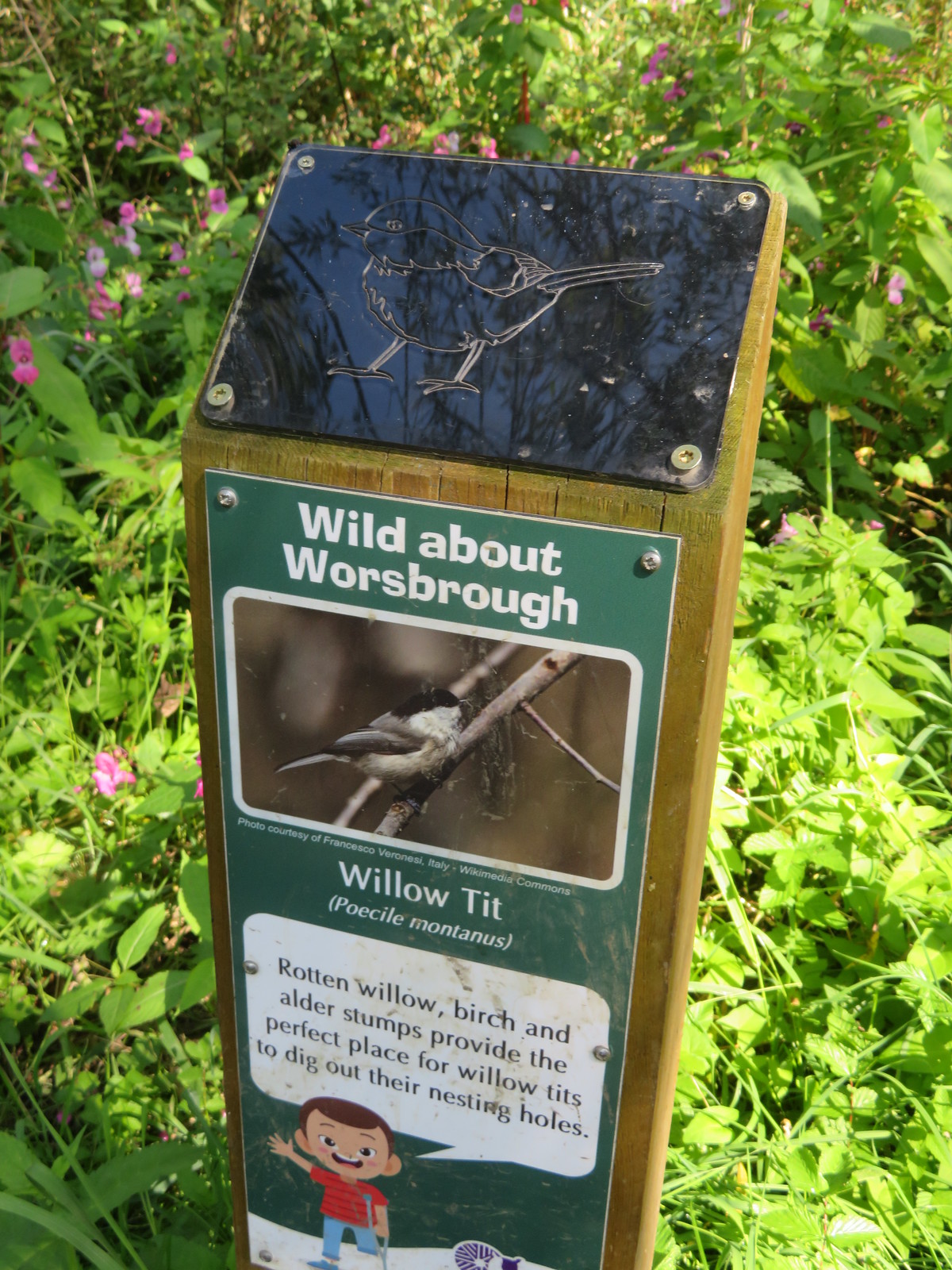The image depicts a detailed informational marker set in a lush garden filled with green plants and some pink flowers. At the top of the wooden post, a dark blue rectangular signboard is secured with screws on all four corners, displaying an outline drawing of a sparrow. Below this, a large vertical green signboard is attached with screws at the top, center, and bottom on both sides. The headline in white letters reads "Wild About Worsbro."

Directly beneath the headline, there is a photograph of a bird perched on a tree branch, enclosed within a white-bordered rectangular box. The text below the photo says "Photo Courtesy of Francisco Veronesi, Italy, Wikimedia Commons." The bird is identified as a "Willow Tit (Poecile montanus)," with the common and scientific names provided. Towards the bottom of this green signboard, there is a cartoon image of a young boy in a red T-shirt, blue pants, and blue shoes. The boy is holding a crutch in one hand and raising the other as if speaking. Next to the boy, in a white speech bubble, is the text: "Rotten willow, birch, and alder stumps provide the perfect place for willow tits to dig out their nesting holes." At the very bottom of the signboard, there is a partially visible purple logo.